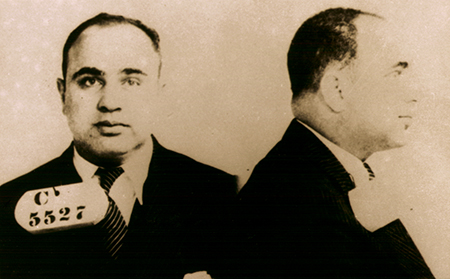The image is an aged, black and white mugshot of infamous gangster Al Capone, presented as a composite of two separate photos merged into one. On the left, Capone is staring directly at the camera, clad in a black business suit, a white undershirt, and a black and white striped tie. A large tag reading "C5527" is visibly pinned to the right side of his suit (the left side of the image). On the right side, Capone is shown in profile, facing to the right, revealing his short hair and balding top. The entire image has yellowed over time, lending a vintage, time-worn quality to the photograph.